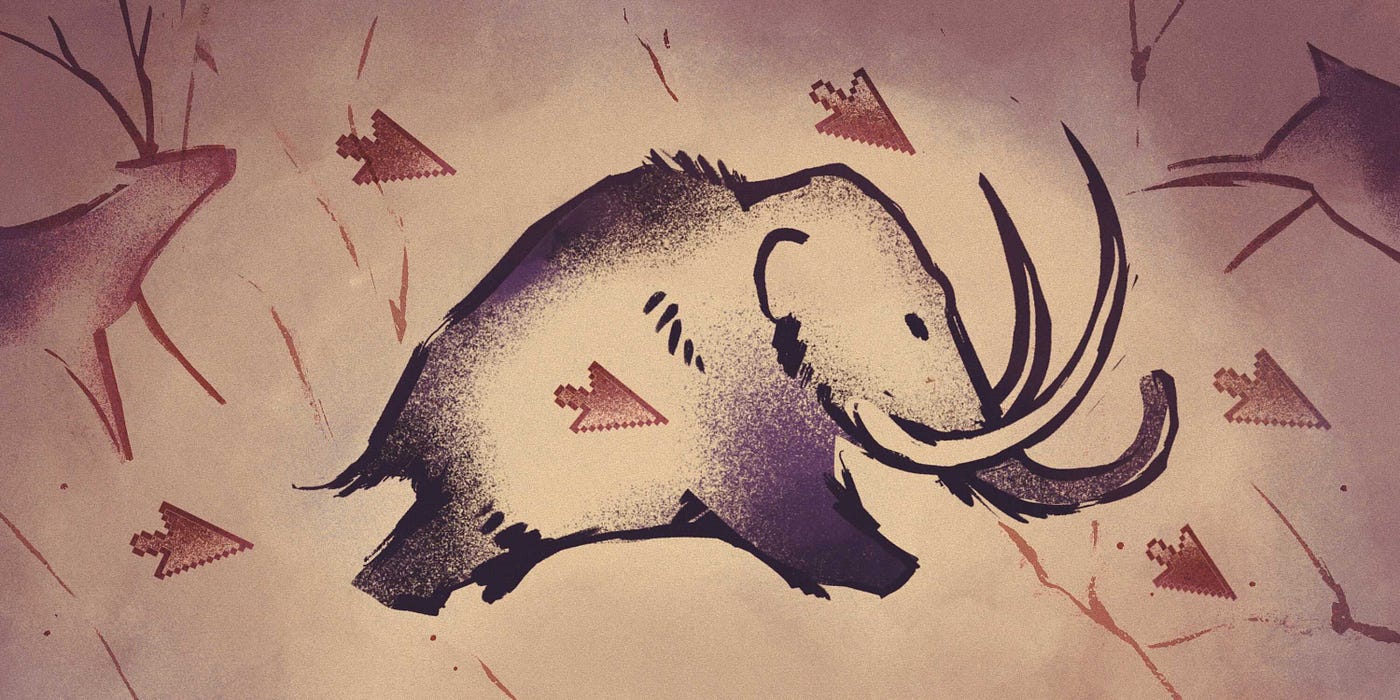The image depicts a prehistoric-style cave painting featuring a central figure, an elephant or mammoth, with long, upward-curling tusks. The elephant, rendered primarily in shades of black, white, and a darker blue that borders on black, dominates the scene with its large presence. The body of the elephant shows a striking contrast with white in the middle and darker hues outlining its form. Surrounding the elephant, there are smaller figures of brown and white deer to its left and right, adding to the primitive atmosphere of the artwork. Red arrows pepper the scene, many pointing in the direction the elephant appears to be moving, with one arrow notably positioned in the center of the elephant itself. The backdrop is a brownish-gray cave wall, and the overall color palette, rich with earthy tones, complements the primitive and abstract quality of the imagery.